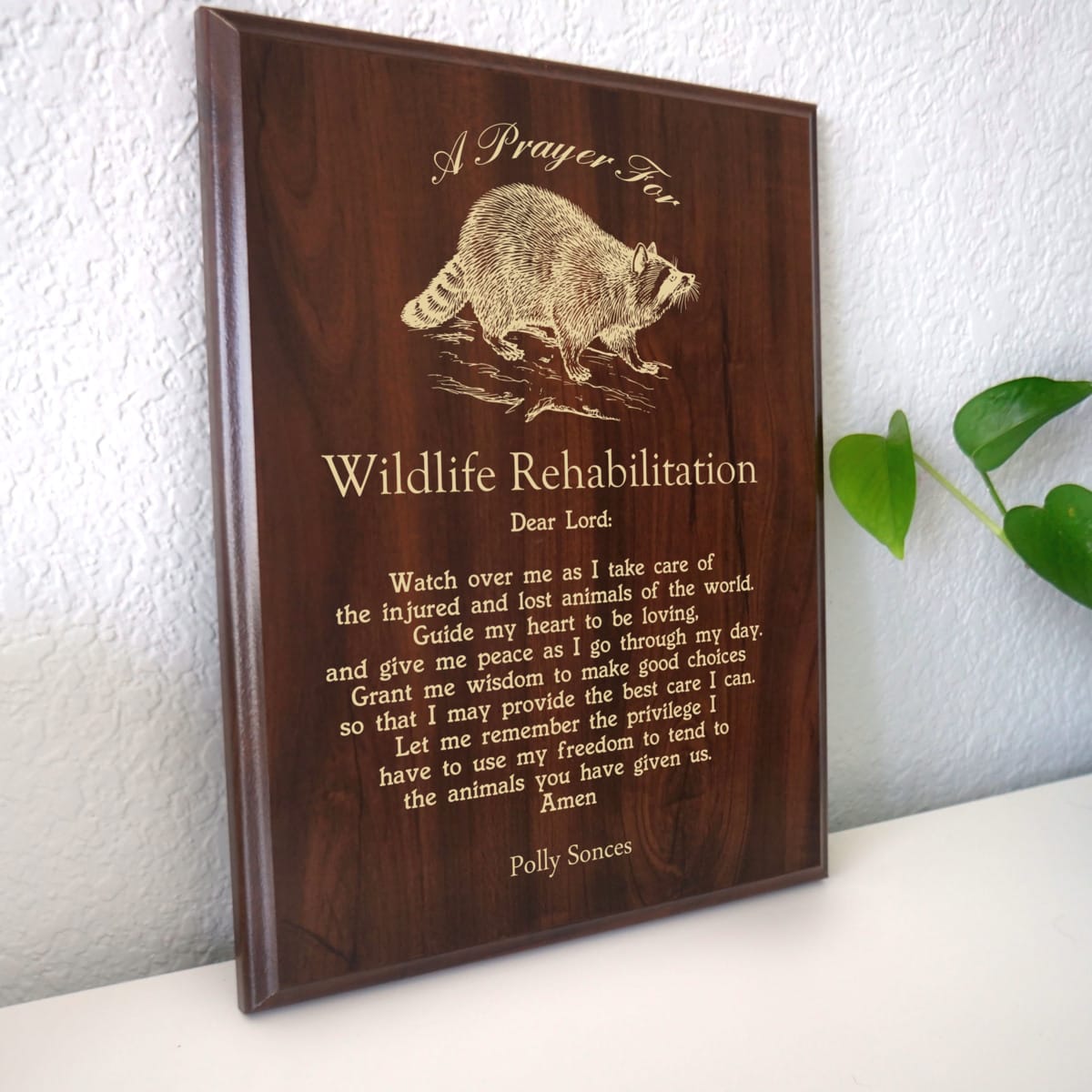The image captures a detailed view of a wooden plaque positioned at an angle, slightly facing to the right, against a white textured wall. This plaque, approximately 12 inches high and brown in color, features an intricately etched raccoon at its center, shaded with dark brown and tan hues. The plaque prominently displays a "Prayer for Wildlife Rehabilitation," penned by Polly Saunce. The prayer reads: 

"Dear Lord, watch over me as I take care of the injured and lost animals of the world. Guide my heart to be loving and give me peace as I go through my day. Grant me wisdom to make good choices so that I may provide the best care I can. Let me remember the privilege I have to use my freedom to tend to the animals you have given us. Amen."

The scene is set on a white tabletop, complemented by three leaves propped up against the wall to the left of the plaque, hinting at a natural theme. Additionally, a small green plant peeks into the photograph from the edge, adding a touch of life and color to the image.